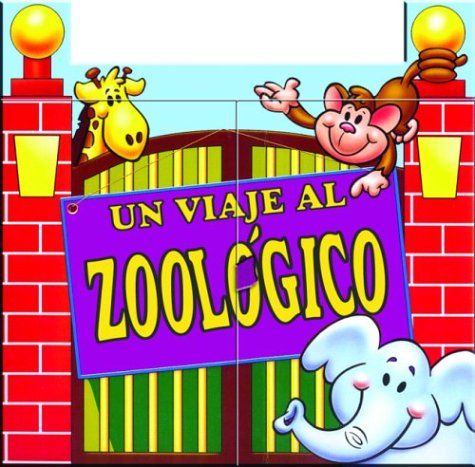This is a colorful cartoon image set at the entrance of a zoo. The scene features a large gate with vertical green and yellow striped bars, framed by narrow, column-like red bricks outlined in white, each topped with a gold ball light. Centered on the gate is a purple sign with yellow letters that reads "UN VIAJE AL ZOOLÓGICO."

To the left of the gate, perched on the brick column, is a smiling giraffe with a yellow face, peeking over the curved top of the gate. To the right of the giraffe, and just to the left of the right-hand brick column, a brown monkey hangs playfully from one of the gold ball lights by its tail, smiling and pointing towards the sign with its left hand. Below, in the bottom right corner, a light bluish-gray elephant with pink spots on its cheeks appears to be smiling, its long trunk curved upward to the right. The background is slightly blue with a white square framing the giraffe and monkey at the top of the image, adding a whimsical touch to this vibrant zoo entrance scene.